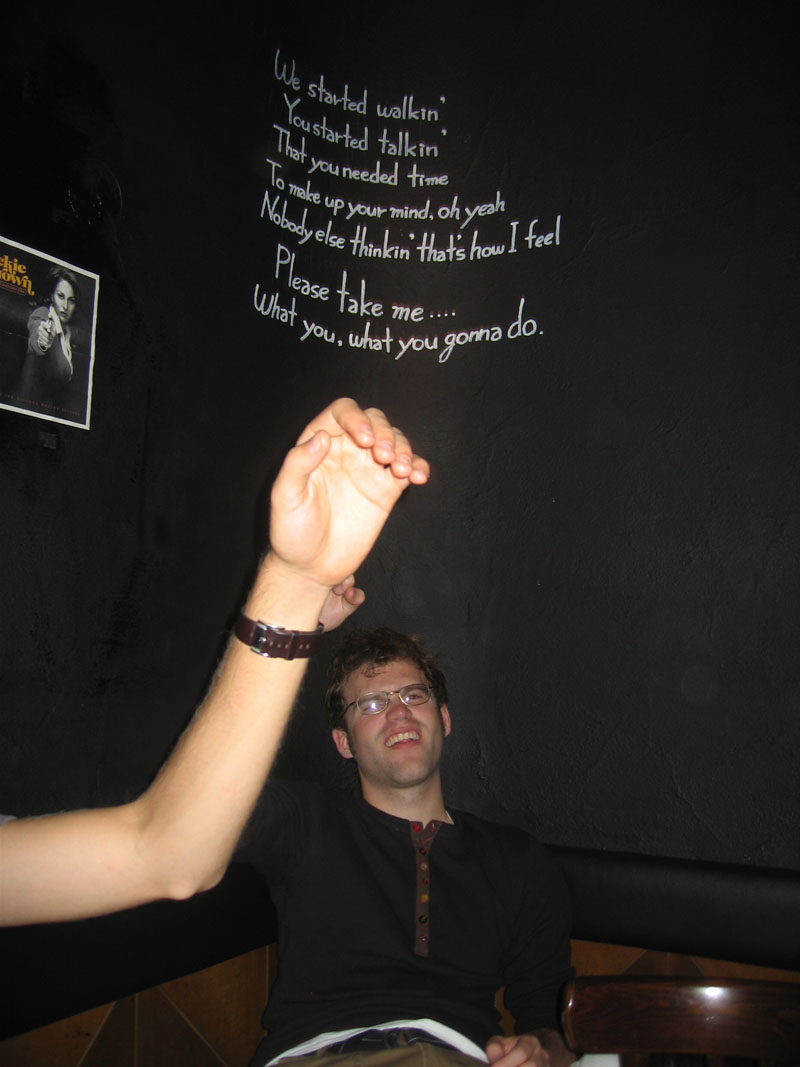In the image, a bespectacled gentleman in a casual dark shirt is sitting in the corner booth of a bar or pub. He has dark hair and is making a perplexed expression while leaning back, revealing the upper row of his teeth. Opposite him, a partially visible arm—adorned with a brown watch—extends into the frame, its hand raised with fingers relaxed. The background features a black wall adorned with white script that reads: "We started walking, you started talking, that you needed time to make up your mind, oh yeah. Nobody else thinking, that's how I feel. Please take me… what you, what you gonna do?" Additionally, a promotional poster for the movie "Jackie Brown" is tacked to the black wall, depicting a woman who appears to be pointing, adding a subtle cinematic touch to the scene. A chair back is visible in the lower right corner of the image.